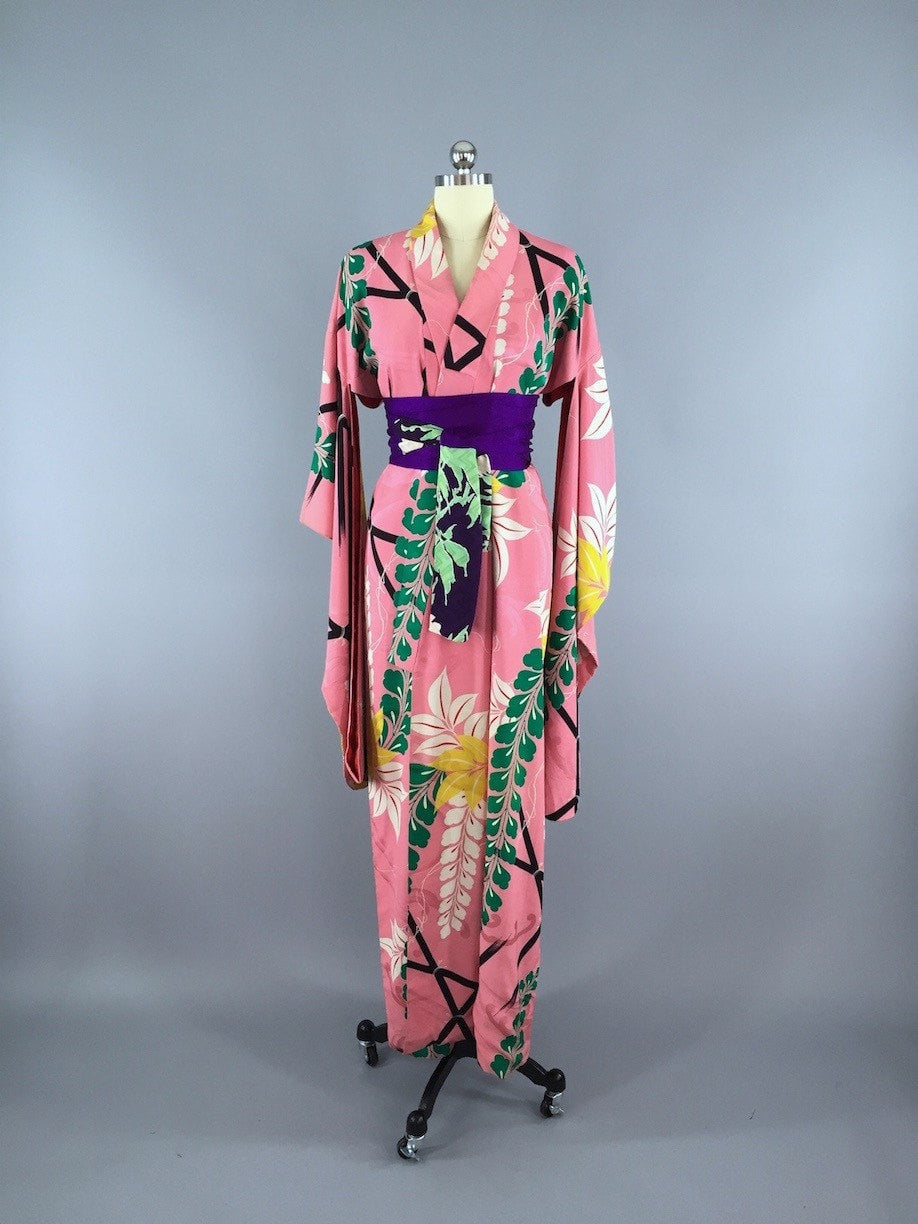The image features a pink kimono draped on a headless mannequin of a white-cream color. The mannequin is mounted on black legs with metallic silver wheels, allowing it to be moved around easily. The scene is set against a gray background, giving it a photo shoot-like atmosphere.

The kimono itself is adorned with a variety of intricate patterns and decorations. There are green leaf vines running along the body and arms, accented by yellow, white, and some red-tinted flowers. Additional white leaves and black lines are scattered throughout the fabric, enhancing its detailed design. A bright purple waistband cinches the kimono at the waist, adding a bold contrast to the overall look. The kimono's long, flowing sleeves and the combination of colors and patterns give it an Oriental, specifically Japanese, aesthetic.